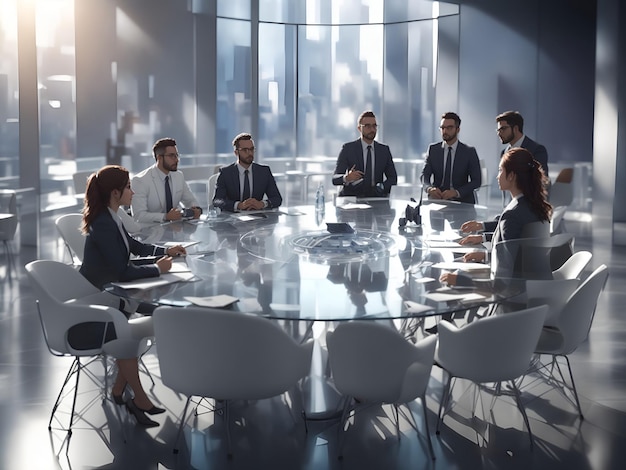The image features a large, round glass conference table surrounded by white chairs, likely made of plastic. Seated around the table are five men and two women, all dressed in business attire. The men are predominantly in dark suits with white shirts and black ties, except for one who stands out in a white suit with a black tie. All the men share similar features, including short dark hair, glasses, and beards. The women, who sit at either end of the table, have long dark hair styled half-up in small ponytails. One wears a dark gray suit with a skirt, while the other is in a light gray suit with a skirt. Each person is holding a pencil with papers in front of them, suggesting they are engaged in a serious discussion. One man in the middle is making a gesture, perhaps emphasizing a point. The background reveals a cityscape visible through large office windows, with light streaming in. This scene evokes the precise and almost uncanny uniformity characteristic of AI-generated imagery.